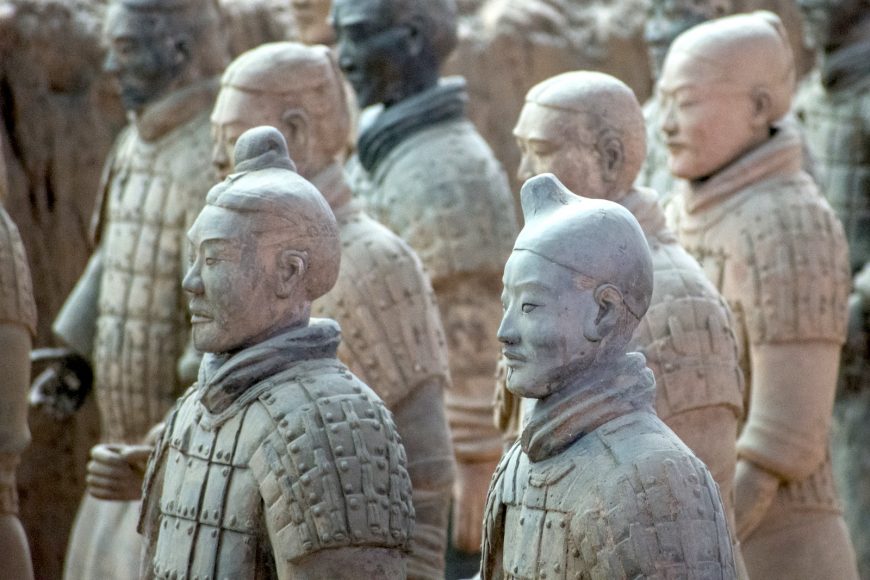The image showcases a group of terracotta statues resembling Japanese military figures. There are likely nine statues visible, with two in sharp focus and the rest slightly blurred in the background. Each statue is adorned in armor, standing in a side view and facing left. The front two statues are distinguished by their intricate details: One has a prominent topknot, while the other's head appears smoother, possibly worn by time, yet still hinting at a former topknot. Both display small goatees, with the statue on the left having an upturned nose, more detailed eyes, ears, and hair, compared to the right statue with a downturned nose and pronounced cheekbones. The garments include armor and large collars, intricately detailed in some statues while worn smoother in others. The statues vary in color from white to tan to very dark shades, evoking a sense of historical grandeur that might be featured in a history channel documentary or magazine, attributable to their detailed craftsmanship and cultural significance.